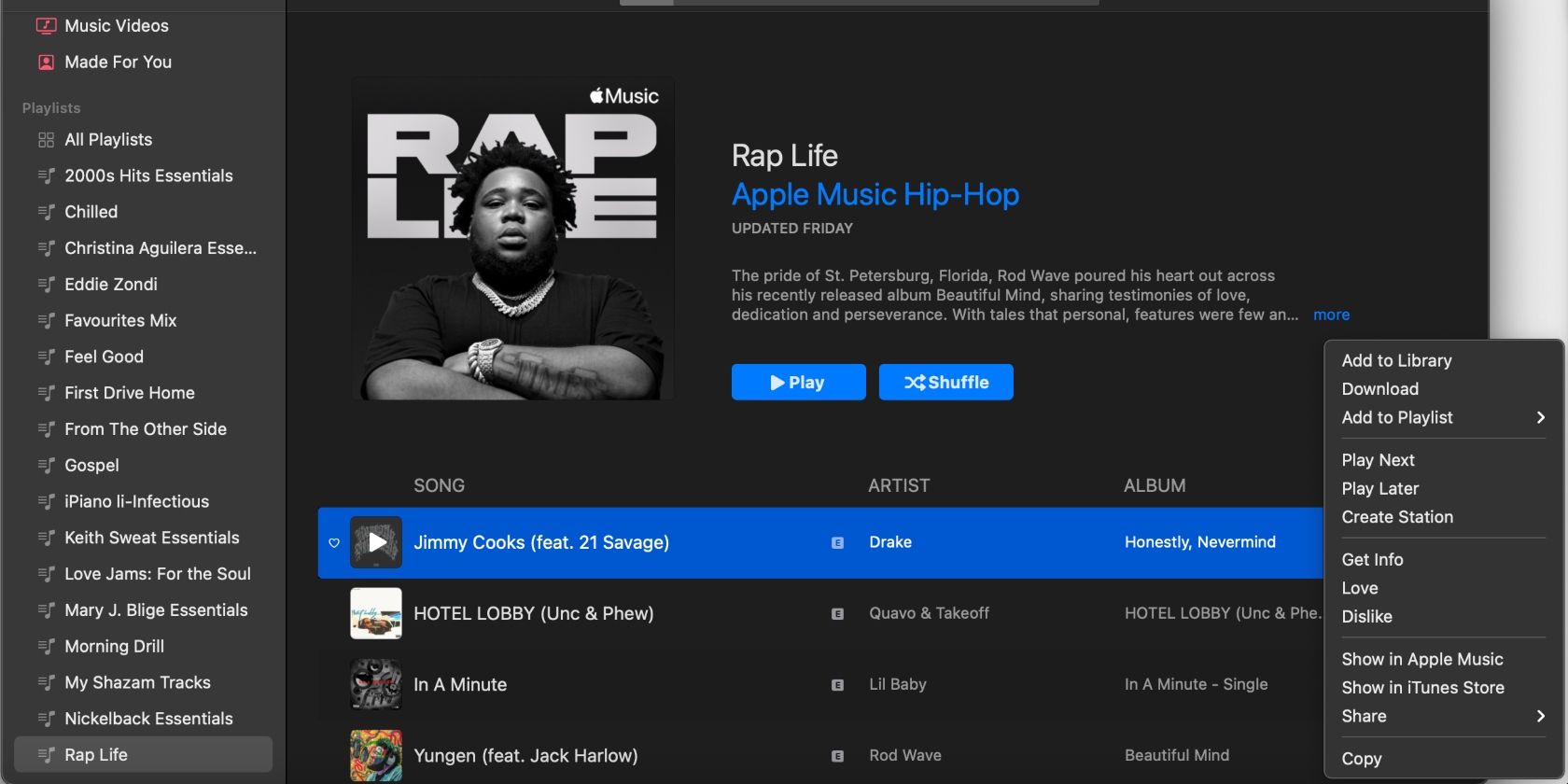This screenshot showcases the Apple Music interface, focusing on a selection of music playlists. The navigation is vertically oriented, with a list of various playlists displayed in gray text. The playlists featured include: "All Playlists," "2000 Hits Essentials," "Chilled," "Christina Aguilera," "Eddie Zondi," "Favorite Mix," "Feel Good," "First Drive Home," "From the Other Side," "Gospel," "iPiano," "Keith Sweat," "Love Jams," "Mary J. Blige," "Morning Drill," "My Shazam Tracks," "Nickelback Essentials," and "Rap Life." Currently, the "Rap Life" playlist is highlighted.

On the right, detailed information about the "Rap Life" playlist is shown. The background of this section is black, with a description of the playlist accompanied by text that says "Apple Music Hip Hop, Updated Friday." There are blue buttons labeled "Play" and "Shuffle" for easy access.

Highlighted in the playlist is the song "Jimmy Cooks" by Drake from his album "Honestly, Nevermind." Various options are available for interaction with this song, including "Add to Library," "Download," "Add to Playlist," "Play Next," "Create Station," "Get Info," "Love," "Dislike," "Show on Apple Music," "Show on iTunes," "Share," and "Copy." Additionally, there are options related to three other artists included in the playlist.